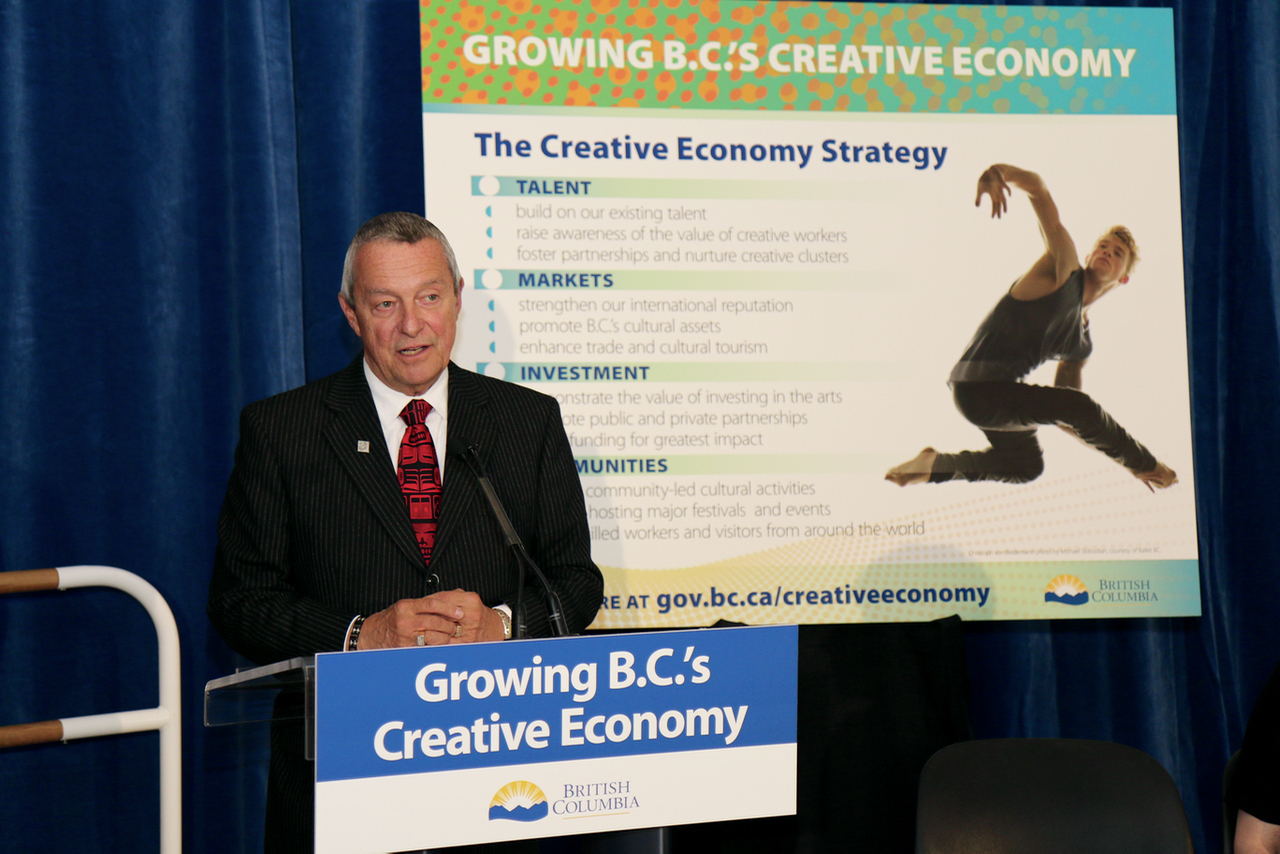In a horizontally aligned rectangular picture, an older man, likely in his 60s, stands at a podium, speaking. He is dressed in a sharp black suit paired with a white shirt and a striking black and red patterned tie, accessorized with a lapel pin and an interesting bracelet on his wrist. His short gray hair has remnants of brown on top, and his mouth is open as if he's articulating a point, with his hands rested on the podium. The podium features a sign that reads "Growing BC's Creative Economy" in white text against a blue background, beneath which is the British Columbia logo on a white background.

Behind him, blue curtains serve as the backdrop for a large square sign that reinforces the theme: "Growing BC's Creative Economy, the Creative Economy Strategy." This sign showcases a male ballet dancer in mid-movement, making an elegant, dynamic pose. Below the main heading, the poster outlines four key areas of the strategy: talent, markets, investment, and communities, with several subset lines under each heading. Part of the text is obscured by the speaker. Additionally, there's a web address listed as gov.bc.ca/creativeeconomy and another British Columbia logo. The overall setting and presentation underscore the focus on developing British Columbia's creative industry sectors.